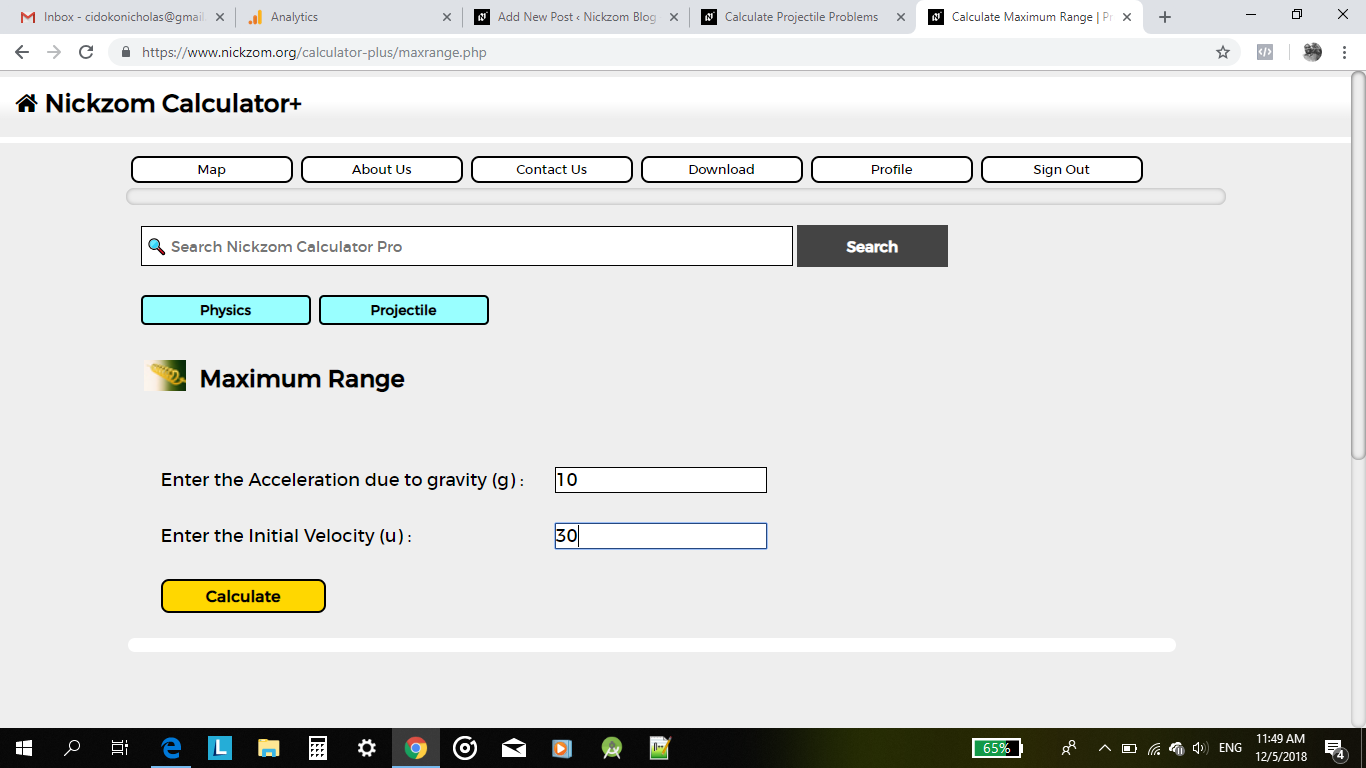A detailed screenshot of a Windows computer screen is displayed, identifiable by the Windows logo resembling a flag or window pane located at the lower-left corner on the Start bar. The browser in use is reminiscent of Chrome but could be a different one. The browser window showcases multiple open tabs, with the fifth tab from the left selected. The tab’s truncated title reads "Calculate Maximum Range | PR".

The URL in the address bar is "www.niczom.org/calculator-plus/maxrange.php". Directly beneath this, the title "Niczom Calculator Plus" is prominently displayed, along with several navigational buttons labeled "Map", "About Us", "Contact Us", "Download", "Profile", and "Sign Out". Beneath the navigation bar, a search field labeled "Search Niczom Calculator Pro" is present, accompanied by a search button.

Further down, two teal buttons with black borders and text are visible, labeled "Physics" and "Projectile". Below these buttons, an image with the title "Maximum Range" is shown. Underneath the image, there are input fields for specific parameters: "Enter the acceleration due to gravity (G):" with an input box displaying the value "10", and "Enter the initial velocity (U):" with an input box displaying the value "30", and the cursor is blinking next to it.

At the bottom, there’s a dark yellow button with a black border and black text, followed by a horizontal line with rounded ends that spans most of the page’s width.